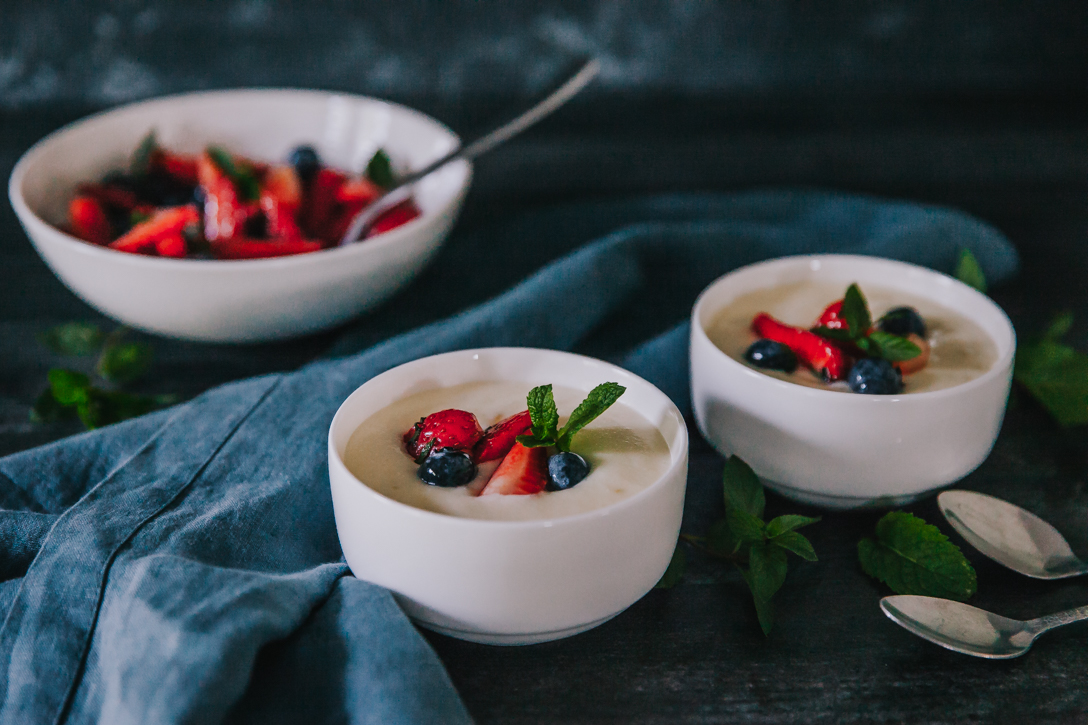The image shows a top-down view of a table adorned with three white bowls and two silver spoons. The upper left bowl, the largest, contains vibrant red and blue fruits—strawberries and blueberries—along with a spoon placed inside. Below and slightly to the right are two smaller, identical bowls filled with what appears to be white yogurt or pudding, topped with the same colorful fruit mix and garnished with mint leaves. In between the bowls, there is a blue towel draped across the table, adding a touch of color. The overall scene has a muted tone, reminiscent of a magazine photo.